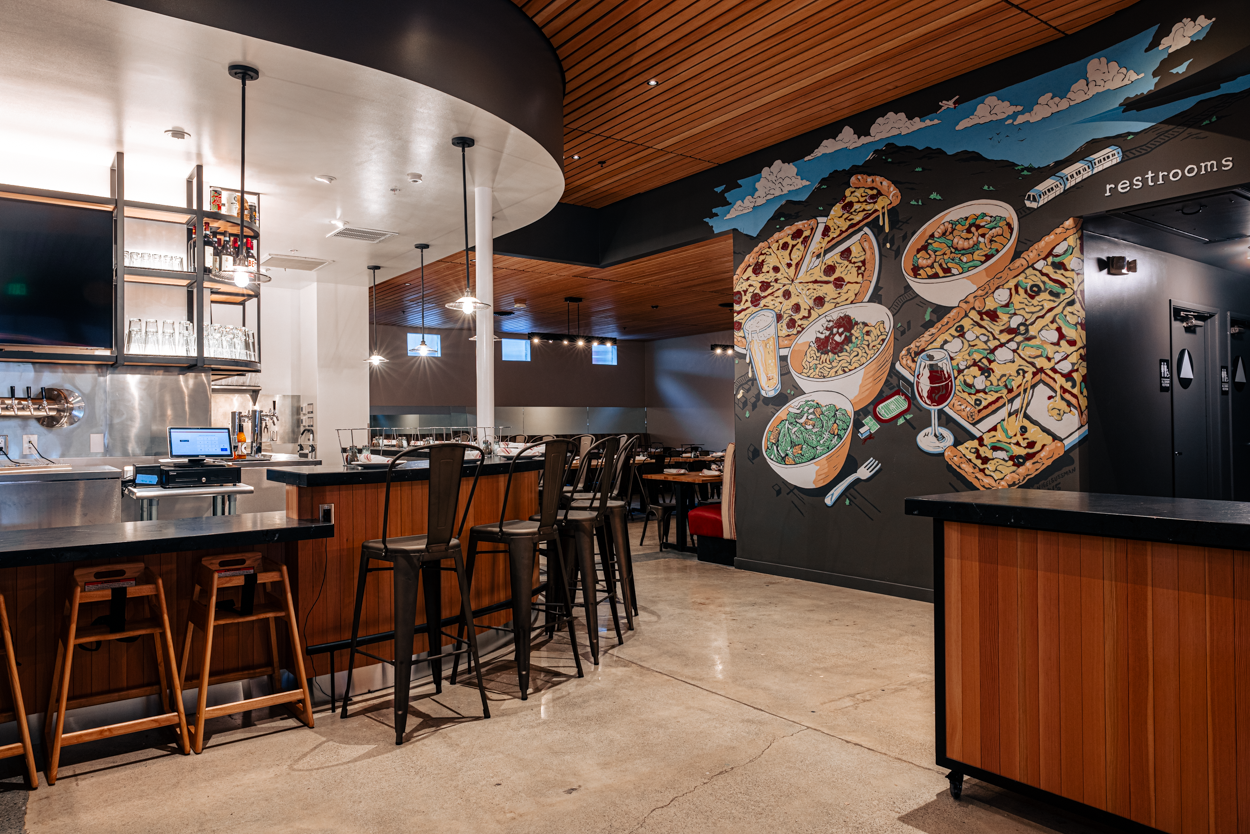The photograph captures a modern, elegant, and updated bar-restaurant interior with a landscape orientation. The scene is viewed from the lobby, focusing on a curved countertop bar on the left, surrounded by black, high bar stools. The bar area is adorned with utensils, cups, laptops, and machinery, and features a computer screen and a big TV. The bar is sleek, with its marble floor, wood grain ceiling, and decorative lighting enhancing its classy ambiance.  

Adjacent to the bar area on the right is a red brick-colored counter with vertical paneling and a black top, leading to an entryway marked by a white sign that reads "restrooms." The doorway is painted dark gray. A large, food-themed mural above the counter showcases various artistic depictions of pizza, salad, pasta, wine glasses, bowls of food, and a rectangular tray of food, rendered in a photographic realism style.

In the background, beyond the bar, is a dining area partially out of view, lit by three windows. The floor is light brown, complementing the wood plank ceiling. The photograph captures the restaurant during a quiet moment, with no patrons in sight, highlighting its refined and contemporary design.